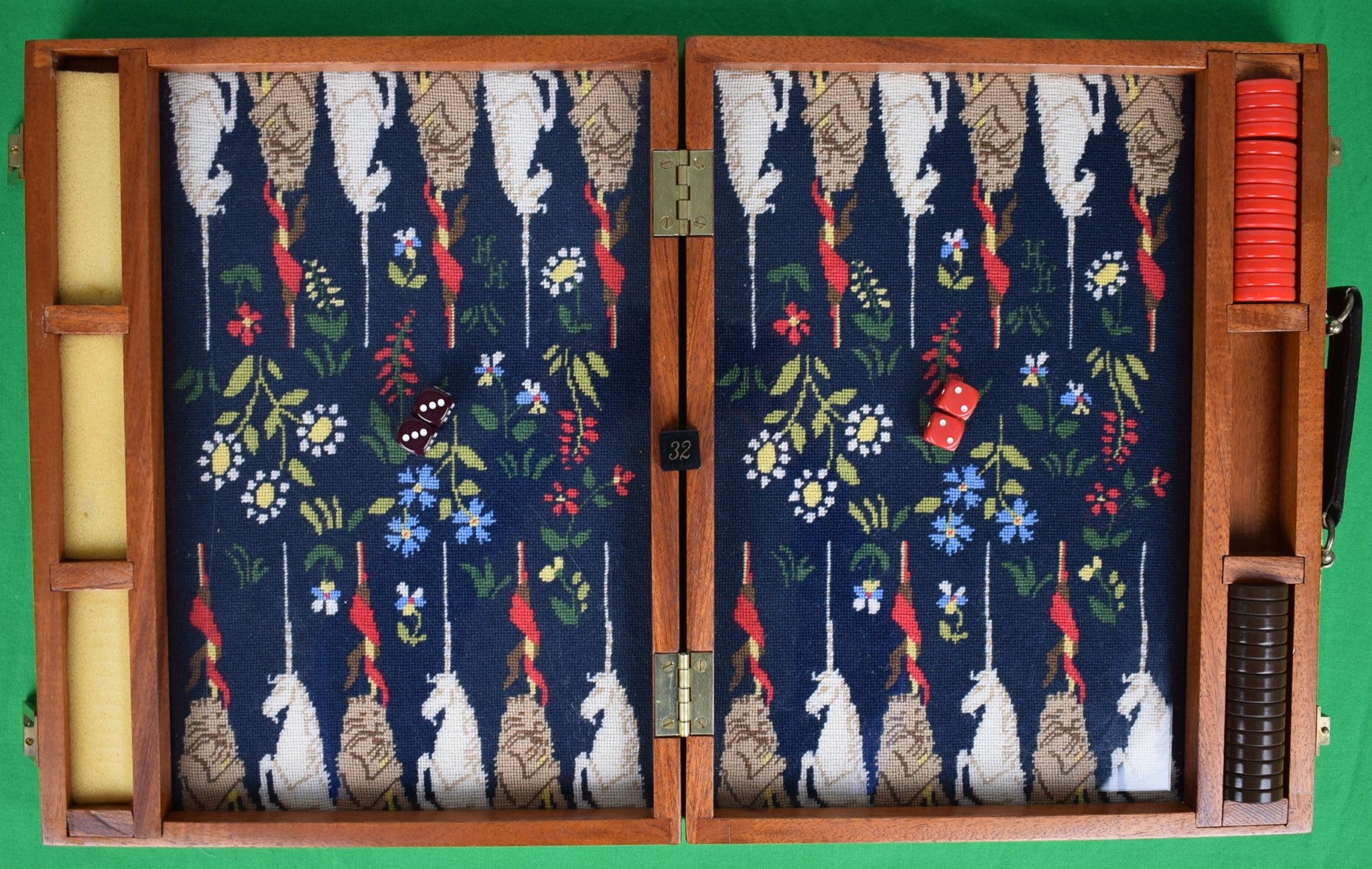This image captures a richly detailed backgammon set presented in an open wooden case, styled like a suitcase with visible hinges in the middle and a handle on the right-hand side. The outer borders of the board are lined with tapestry-like fabric featuring alternating patterns of brown and white unicorns where the pips typically would be. The middle sections of both halves of the board are adorned with vibrant floral designs showcasing blue, red, yellow, white, and green flowers on a navy felt background.

The right side of the board displays three segments; the top segment contains lined-up red backgammon pieces, the middle is empty revealing the wood frame, and the bottom segment holds the black playing pieces. On the same side, a pair of red dice shows two dots each.

The left side mirrors the right but with black dice, each displaying three dots. The whole frame, a piece of craftsmanship, is constructed from high-quality wood and includes small black metal hardware, with one piece marked with the number 32. This ornate set not only serves its purpose for play but stands as a beautiful piece of functional art.